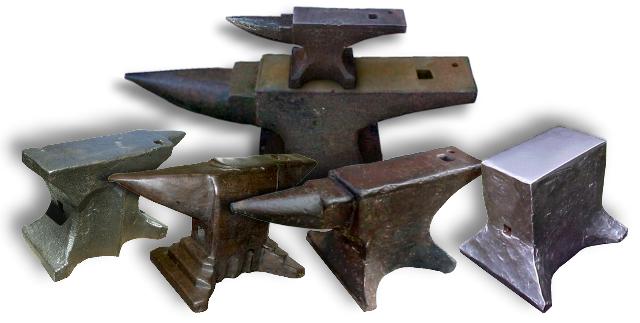The image depicts six anvils of varying sizes and designs arranged on a digitally-simulated white background. In the foreground, there are four anvils lined up from right to left. The two central anvils share a similar design with a slight difference in their base stands. The anvil positioned on the far right is a distinctive silver cube with legs, unlike the others, and lacks the characteristic horn shape. The anvil on the far left is darker, resembling iron. Additionally, at the back of the display, there are two larger anvils, with the smaller one stacked on top of the larger. Most of the anvils exhibit a worn, bronze-rust finish, except the silver cubic anvil. The simulated white background and shadows suggest the anvils are digitally presented, emphasizing their unique forms and utilitarian design for metalworking.